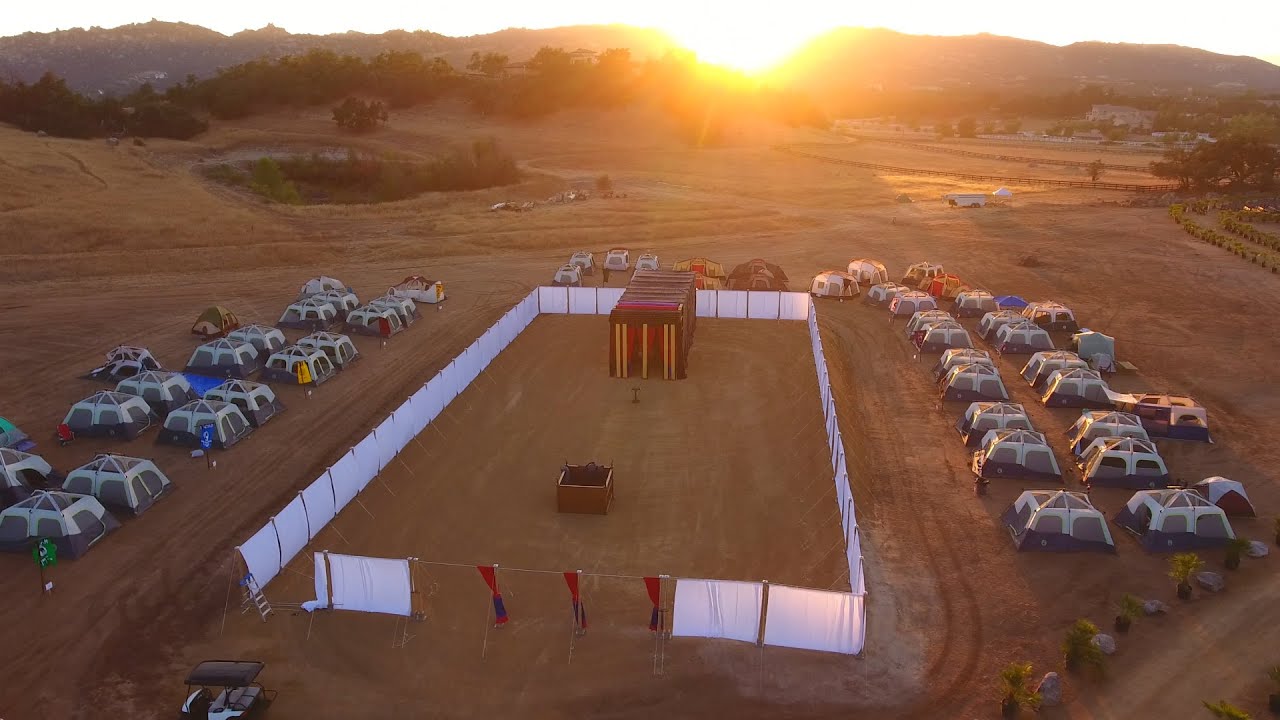This aerial image showcases a desert scene resembling an outdoor festival or biblical tableau, set against the picturesque backdrop of a sun setting behind distant hills and mountains. Central to the composition is a large, rectangular enclosure formed by white sheets, which serves as a barrier. Inside this enclosure, on one end, there's a vibrant, flat-roofed red tent adorned with yellow-striped curtains. On the opposite end, a hollow, brown box structure with red and yellow accents stands out.

Surrounding this central area, there are numerous modern dome tents, mostly gray with white accents, interspersed with a few different styles of tents. Each tent is marked by colorful flags, including green, red, blue, and yellow. A sizable group of these tents is positioned to the left, back middle, and right of the enclosure.

In the broader scene, there's a dirt-covered ground with visible trails and a road running to the right. A golf cart is situated in the front left of the image. The distant background features an oasis with trees and an established community of white buildings, adding depth and a sense of place to the overall landscape.